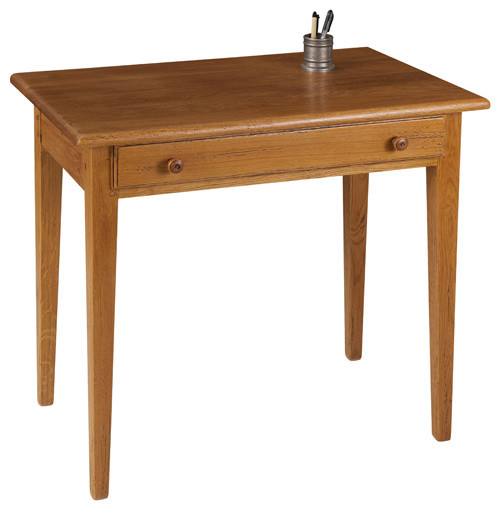In this close-up image, set against a completely white background, we see a small, medium brown, maple desk positioned directly in the center at a diagonal angle. The desk has a rectangular top with a silver pencil holder in the upper right corner containing pens and pencils. Beneath the top, there is a single drawer accented by two widely spaced knobs, suggesting ample storage space. The desk is supported by four slender, straightforward legs. This minimalist and elegant piece could easily fit into a website catalog for furniture, given its simple yet functional design.